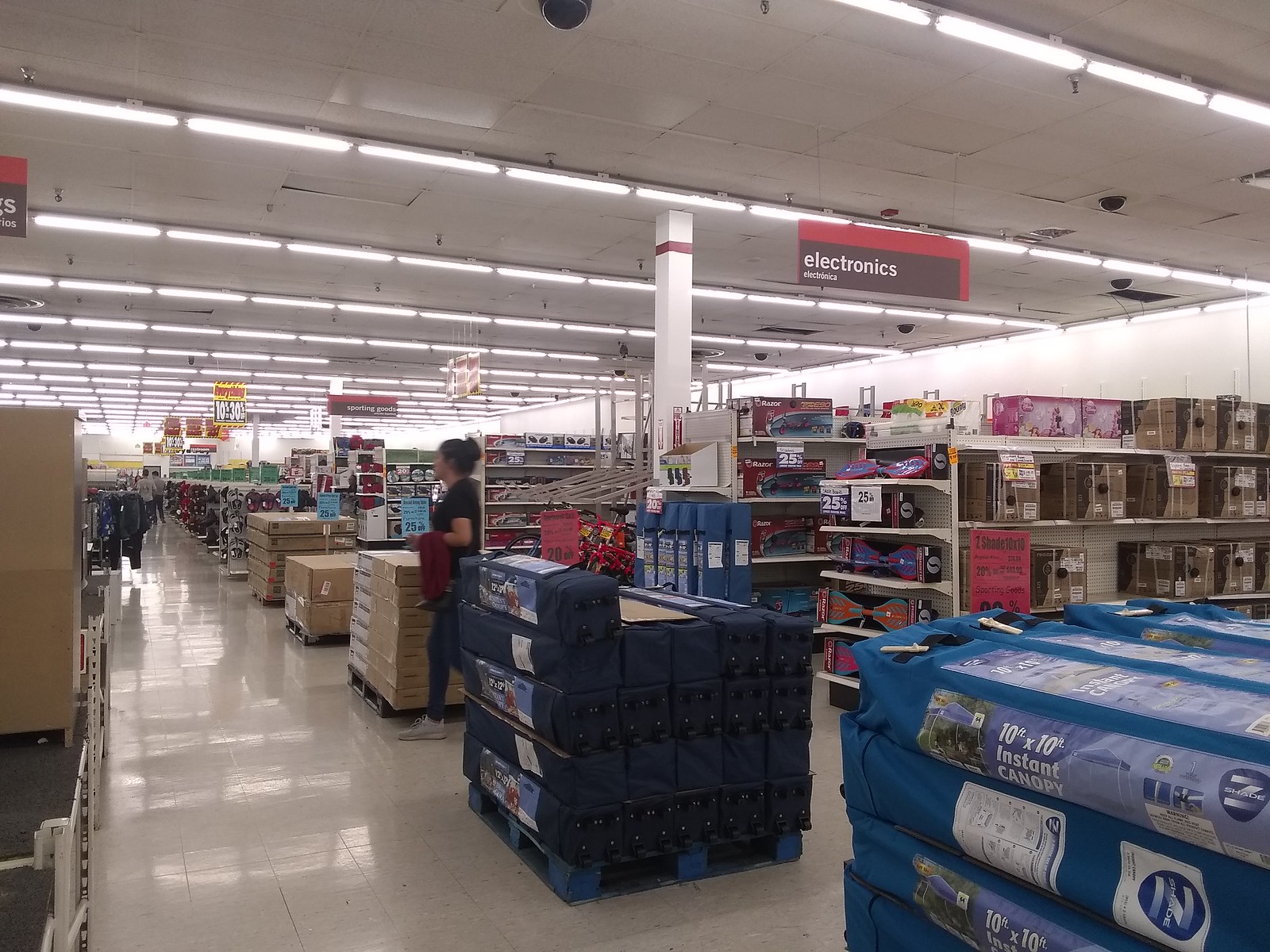This color photograph captures the bustling interior of what appears to be a large superstore, possibly a Target, adorned with white tile ceilings and rows of fluorescent track lighting. The store's right-hand side showcases aisles with fully stocked shelves, though the exact items are indistinguishable from the distance. A prominent gray sign reading "Electronics" hangs from the ceiling, adding to the structured layout of the space.

In the foreground, there are two large palettes of stacked items. The nearest palette carries blue, 10x10 instant canopies, arranged in piles about four to five high and across. Slightly further back, another palette, roughly four to five feet away, holds dark blue items, which could be tents or another type of canopy. The floor is a gray-beige tile, extending through the aisle.

Centrally placed in the scene is a woman walking from right to left. She has dark hair tied in a knot and is attired in a short-sleeved black shirt, blue jeans, and gray shoes, while holding a red sweater or hoodie. Her pale complexion is just discernible from the distance at which she is photographed. The background is filled with an array of indistinct merchandise on shelves, aligned in precise rows, emphasizing the store’s extensive inventory and organized structure.